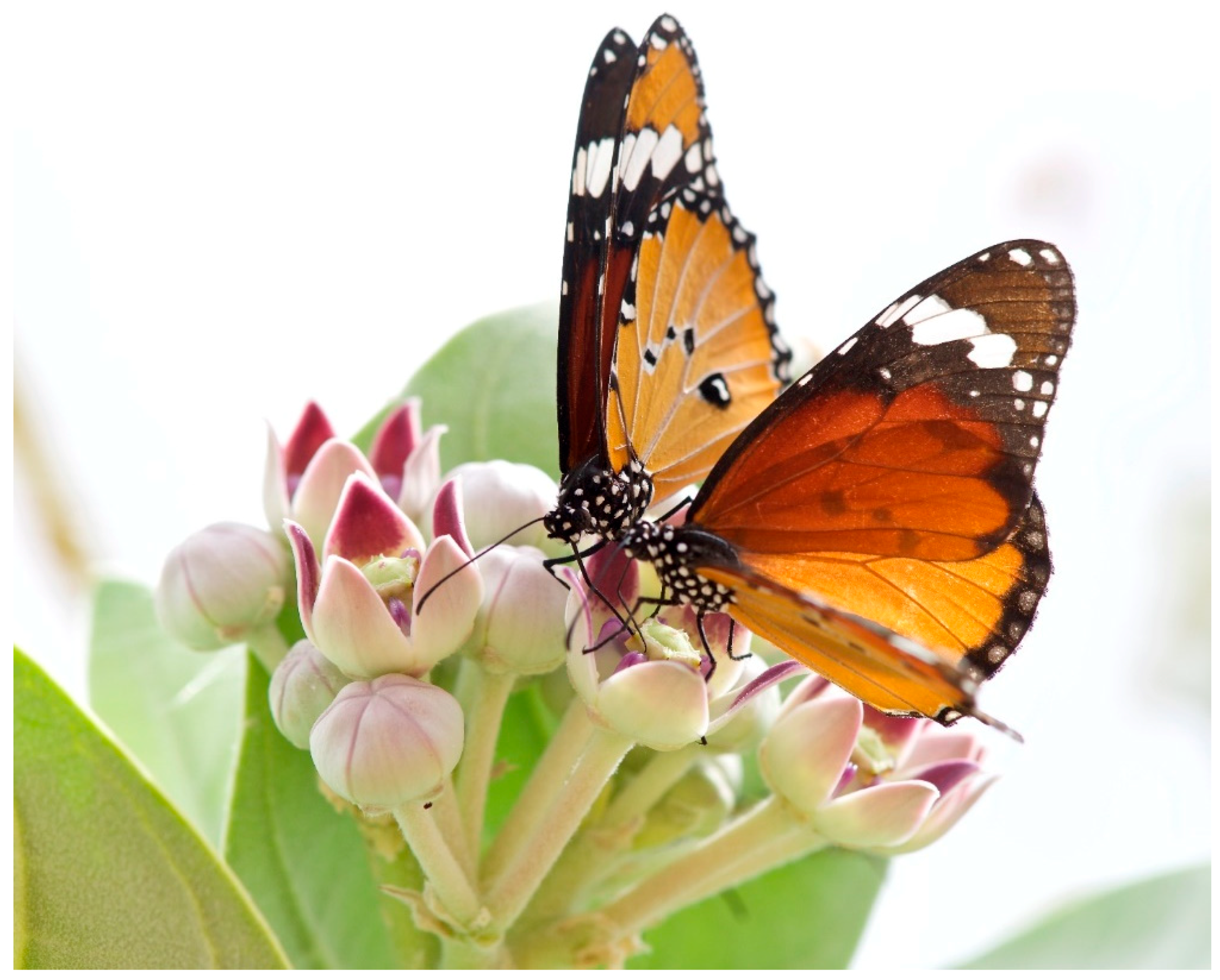The image is a vibrant, professional nature photograph taken outdoors on a sunny day using natural light. It is a square, full-color close-up shot, with an indeterminate white background occupying the upper portion and right side, adding a minimalistic contrast that highlights the subject.

In the bottom left corner, green leaves rise up rather than hanging down, adorned with white flowers that display shades of reddish-pink on the inside and green pollinated centers. The flowers are in various stages of blooming; some remain closed, while others are beginning to open.

Perched atop these flowers are two monarch butterflies, positioned very close to each other, almost touching. Each butterfly is characterized by its predominantly orange wings bordered in black with white spots, and a black body also speckled with white. The intricate patterning on their wings includes black spots with white centers amidst the vibrant orange. The detailed capture emphasizes the delicate beauty of the butterflies and the intricate forms of the partially blossomed flowers.